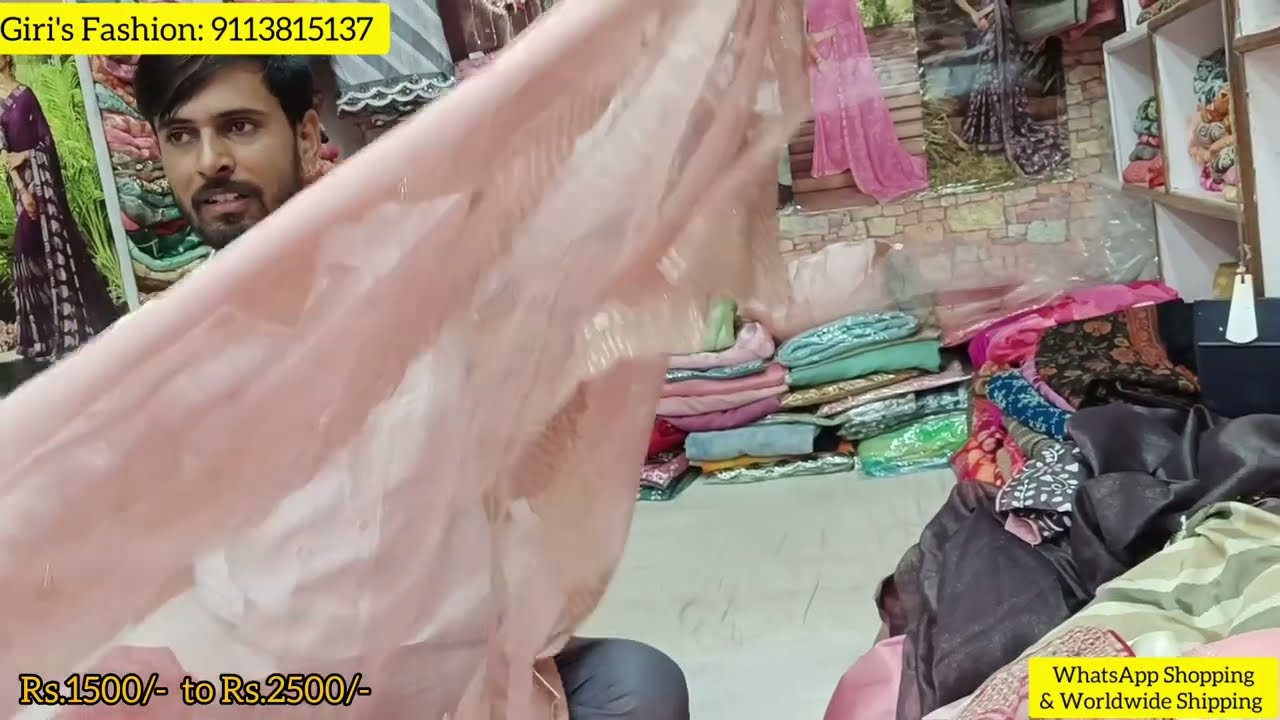In this image, we see a vibrant scene that appears to be from a fabric store or market, specializing in clothing and accessories. A young man with dark hair, who looks to be of Indian ancestry, is prominently holding up a large, silky piece of bright pink fabric, showcasing it to potential buyers. The background behind him is filled with stacks of folded fabrics in a multitude of colors such as greens, pinks, and blues, along with various accessories, suggesting a rich variety of merchandise.

In the upper left corner of the image, within a yellow rectangle, it reads "Girls Fashion; 9113815137" in black text. This indicates the store's contact information, possibly for orders or inquiries. Additionally, another yellow rectangle in the bottom right corner announces, "WhatsApp Shopping and Worldwide Shipping," also in black text, highlighting the store's offer of global shipping and a convenient shopping method via WhatsApp.

Furthermore, the image contains a pricing detail in a smaller text found below the advertised fabric: "RS 1500 to RS 2500," suggesting a range of prices for the products available. This detailed signage and the man's active display of the pink fabric point towards a bustling environment where customers are invited to explore and purchase various colorful fabrics and fashion items.